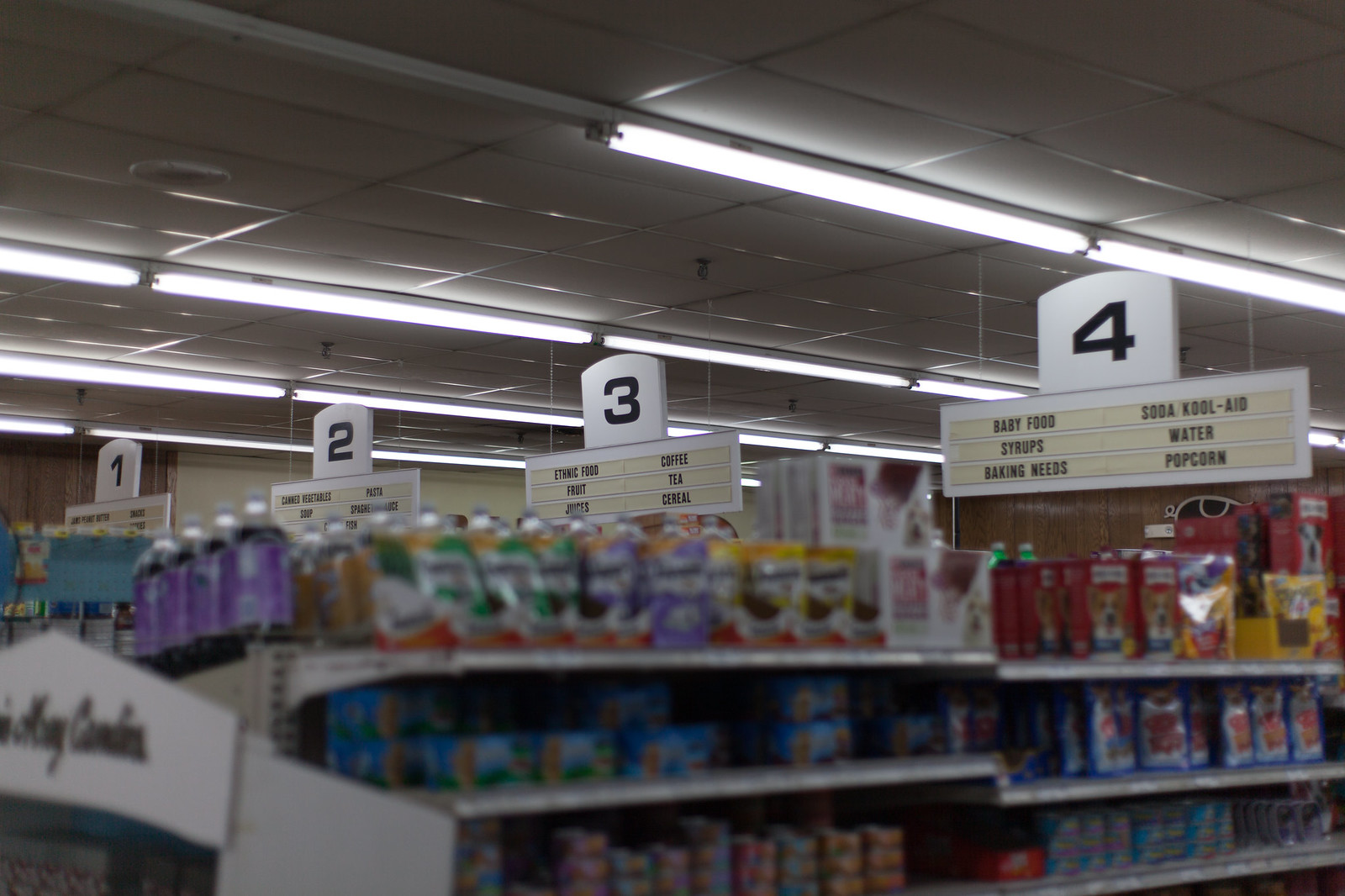The image depicts the interior of a grocery store, showcasing four visible aisles. The most prominent aisle, marked as Aisle 4, is stocked with various cans of pet food, although the text on the cans is somewhat blurred. Adjacent to Aisle 4, another part of the same aisle sign lists several categories of products including baby food, syrups, baking supplies, soda, Kool-Aid, water, and popcorn.

Aisle 3 displays a sign indicating the presence of ethnic foods, juices, coffee, tea, and cereal. Although Aisles 1 and 2 are not clearly visible in the image, their vague outlines hint at their existence. The ceiling features long, possibly fluorescent light fixtures and appears to have a drop ceiling design, providing ample illumination to the well-stocked and organized aisles below.